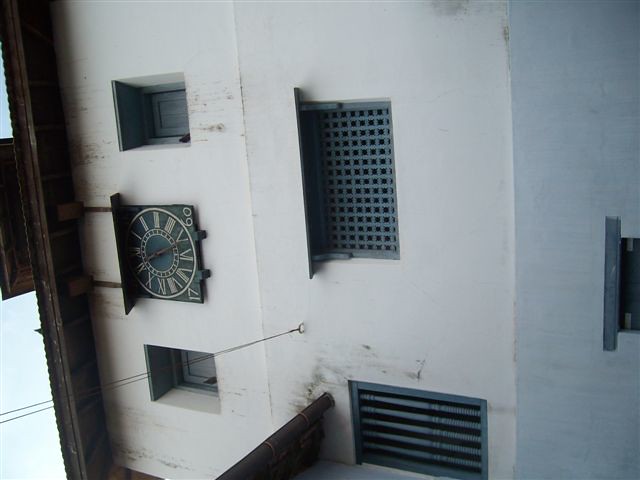The image depicts a sideways view of an old, white building that appears worn and dirty. Prominently visible are two windows towards the bottom, each covered with bars—one with horizontal bars and the other with a grid of intersecting horizontal and vertical bars forming small squares. The building features several window cutouts—five full ones and a sixth partially visible on the right margin. Among these cutouts, the top left reveals a plain green background, while the second from the top showcases a green clock with gold Roman numerals and brown hands, partially obscured by the angle. Below the clock, there is a plain white box. The central cutout displays a vertically-oriented, graded green rectangle, and the bottom cutout features green horizontal bars.

The building's roof appears to be made of slate and there is a protruding box or awning above the clock. The clock itself, dated 1760, is mounted on the building’s exterior, hanging from two brackets, with wires attached to a hook beneath it. Outside, there's a table-like structure with a high, straight platform. The overall scene conveys an impression of age and neglect.